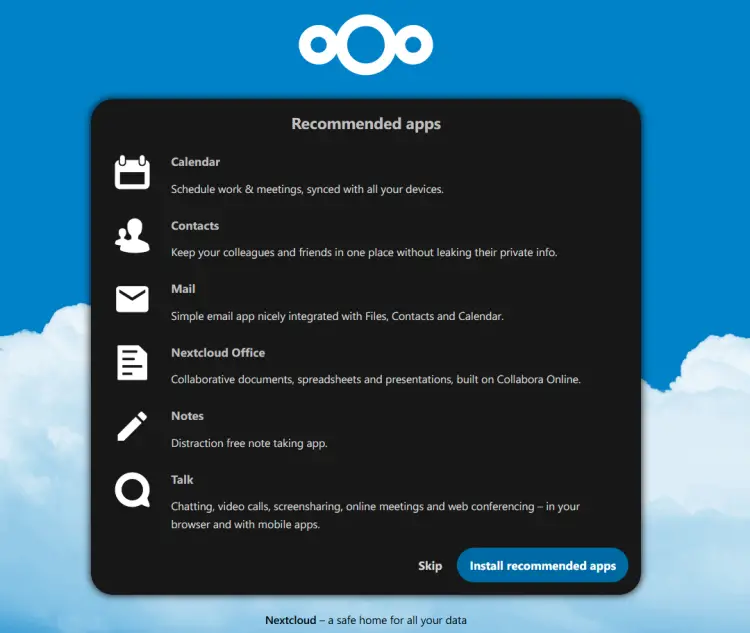The image is a screenshot featuring a clean interface against a backdrop of clouds and a clear blue sky. At the top center, three circles form a logo. Below, a central black background with white text is prominently displayed. The heading reads "Recommended Apps," followed by a list of six app suggestions, each accompanied by an icon and description.

1. **Calendar Icon** - 'Schedule' app: Manage work and meetings seamlessly across all your devices.
2. **User Icon** - 'Contacts' app: Keep colleagues and friends organized while safeguarding their private info.
3. **Mail Icon** - 'Mail' app: An easy-to-use email client well-integrated with your files, contacts, and calendar.
4. **File Icon** - 'NextCloud Office': Collaborate on documents, spreadsheets, and presentations with Calibora Online.
5. **Pencil Icon** - 'Notes' app: Enjoy distraction-free note-taking.
6. **Magnifying Glass Icon** - 'Talk' app: Engage in chatting, video calls, screen sharing, online meetings, and web conferencing directly in your browser and via mobile apps.

At the bottom of the screen are two options: a "Skip" button and a more prominent blue button labeled "Install Recommended Apps" in white font.